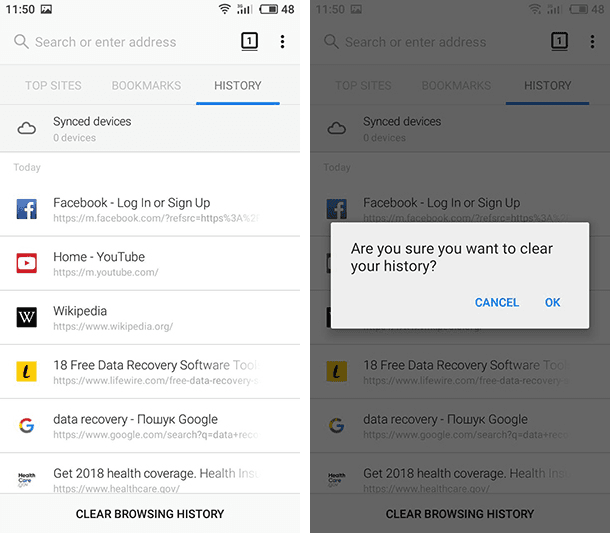Here's a detailed and cleaned-up caption for the image:

"Screenshot of a smartphone browser displaying the history tab. The phone on the left shows a timestamp of 11:50 and a battery level at 48%. At the top, there's a search bar to enter an address, showing an icon with the number '1'. Below, the browser tabs include 'Top Sites,' 'Bookmarks,' and currently selected 'History.' The 'Synced Devices' section shows zero devices. In the browsing history, several entries are listed, each with corresponding logos: 

1. Facebook (Log In or Sign Up)
2. YouTube (Home)
3. Wikipedia
4. A special site about '18 Free Data Recovery Software Tools'
5. Google
6. Another data recovery link, with the first word written in Cyrillic
7. A site for 2018 Health Coverage and Health Insurance

At the bottom, there is an option to 'Clear Browsing History.' The phone on the right displays the same screen but with a pop-up overlay. The background is greyed out, and the white pop-up reads 'Are you sure you want to clear your history?' in black text. At the bottom of the pop-up, there are two blue buttons: 'Cancel' and 'OK,' indicating that the user can confirm or cancel the action of clearing the browser history."